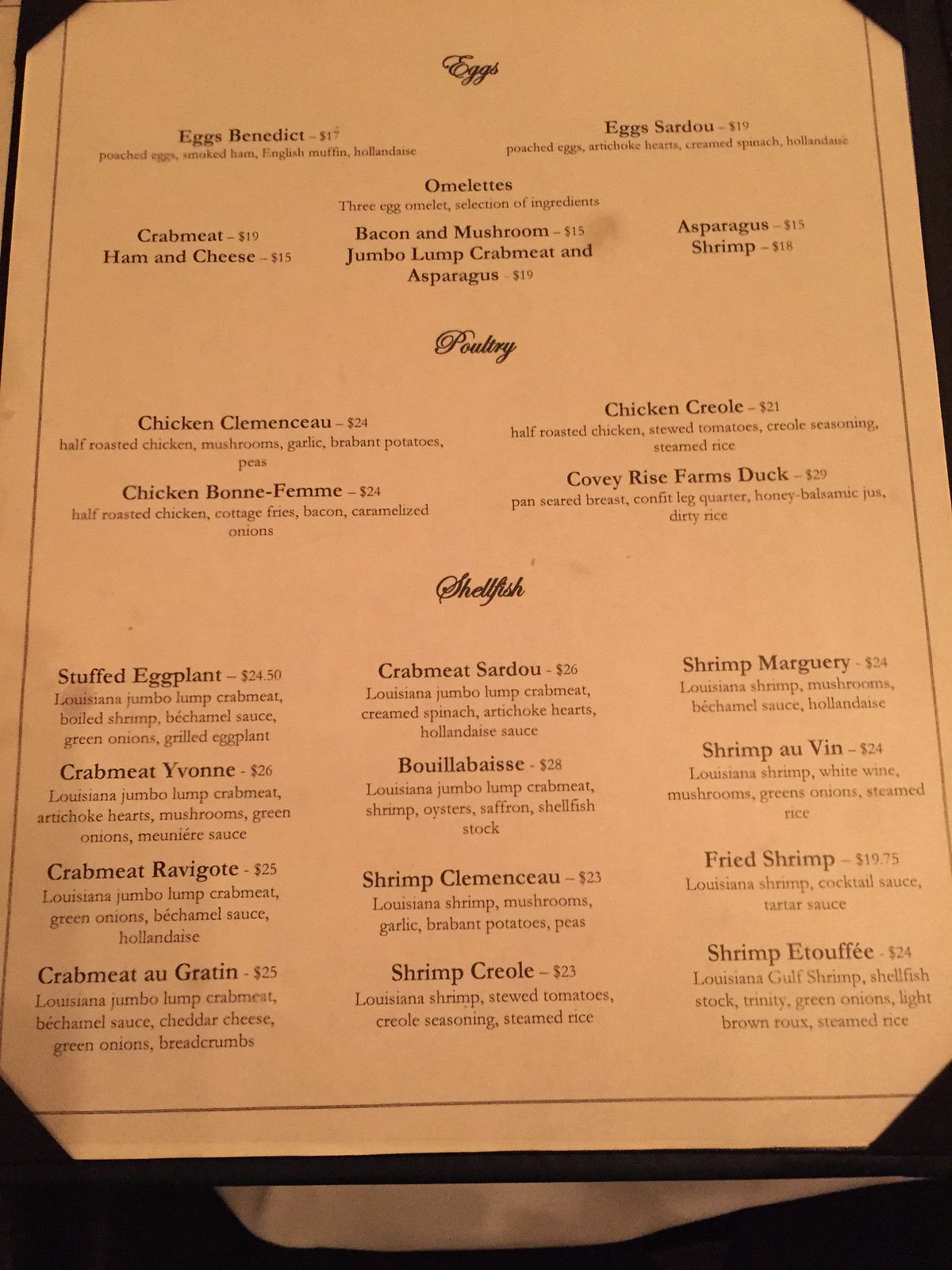**Detailed Breakfast Menu Description**

This image captures a top-down view of a breakfast menu, taken with a camera or phone rather than being a scanned copy. The white table surface is slightly visible at the lower part of the image, indicating the setup.

The menu itself appears to be a light-colored piece of paper, possibly white with a pinkish hue due to the lighting or camera settings. It is neatly tucked into a black cover at all four corners, giving it a sophisticated, hardback menu look.

The content of the menu is as follows:

- **Title**: Eggs
  - **Left Column**:
    - Eggs Benedict - $17
    - Eggs Sardou (with descriptions for each dish below)

- **Sub-section**: Omelets
  - **Left Column**:
    - Crab Meat
    - Ham and Cheese
    - Bacon and Mushroom
    - Lumberjack
  - **Right Column**:
    - Crab Meat and Asparagus
    - Asparagus and Shrimp
    
- **Section**: Chicken & Poultry
  - **Left Column**:
    - Chicken Clemenceau
    - Chicken Creole
  - **Right Column**:
    - Chicken Bonne Femme
    - Covey Rise Farm Duck

- **Section**: Shellfish
  - The shellfish section is organized into four rows and three columns of dishes.
  - **First Column**:
    - Stuffed Eggplant
    - Crab Meat Yvonne
    - Crab Meat Ravigote
    - Crab Meat au Gratin
  - **Second Column**:
    - Crab Meat Sardou
    - Boula Boula
    - Shrimp Coleslaw
    - Shrimp Creole
  - **Third Column**:
    - Shrimp Marigny
    - Shrimp Bellevue
    - Fried Shrimp
    - Shrimp Étouffée

This layout provides a comprehensive overview of the various breakfast options available, ranging from egg dishes and omelets to chicken, poultry, and an extensive selection of shellfish dishes.